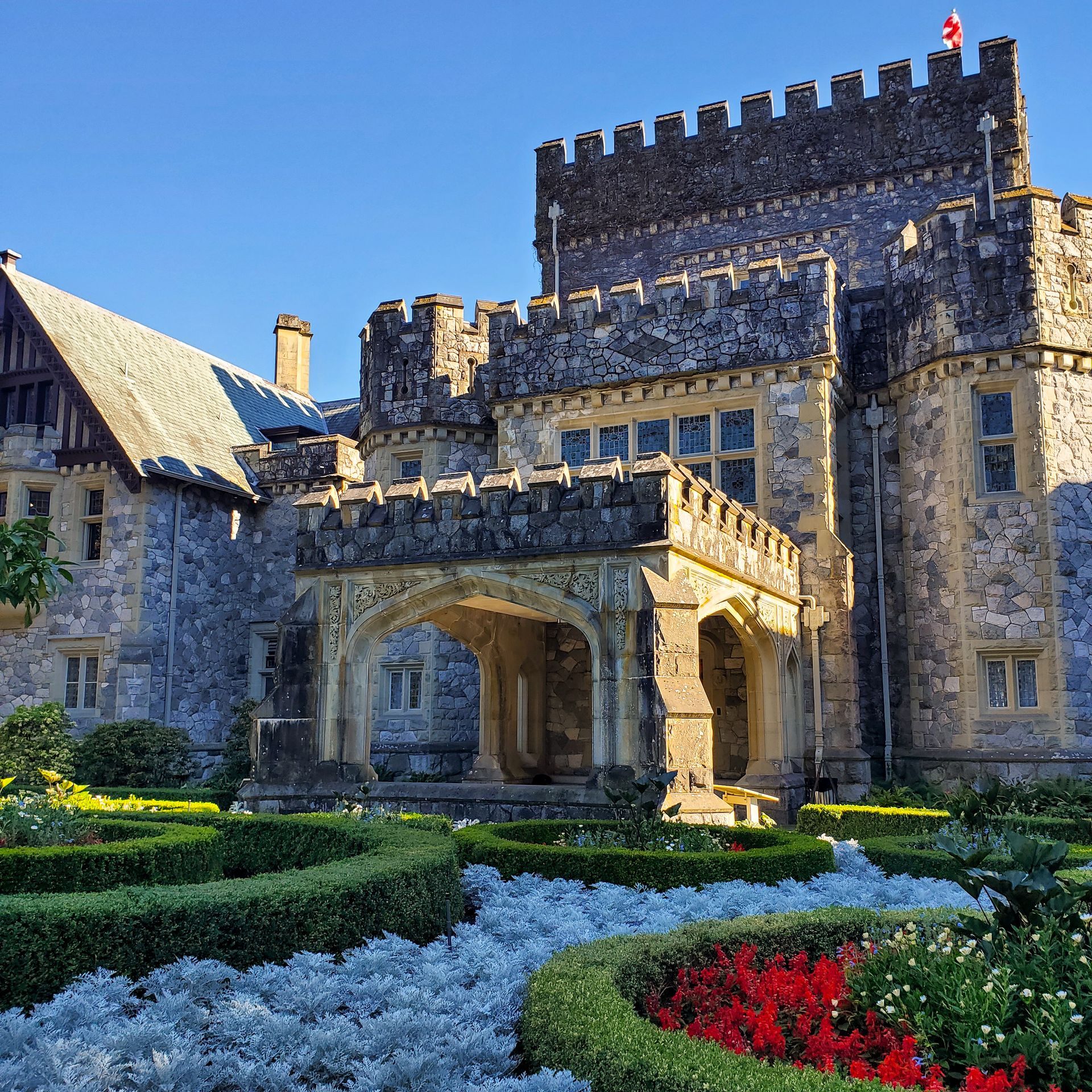The photograph showcases a grand modern castle, its impressive architecture standing prominently against a meticulously maintained landscape. The spacious grounds in front of the castle are thoughtfully designed with distinct sections. In the center, desert-type plants, which seem slightly out of place amidst an array of vibrant red and white flowers, add an intriguing contrast. Circular hedges neatly divide these floral areas, perhaps representing elements of water in their design. The castle itself features a layered structure starting with a low-roofed entrance area, leading up to another elevated section, and culminating in a three-level watchtower. To the left, a small housing area is visible. At the very top of the castle, a flag featuring red and white colors with an emblem resembling an eagle waves proudly.